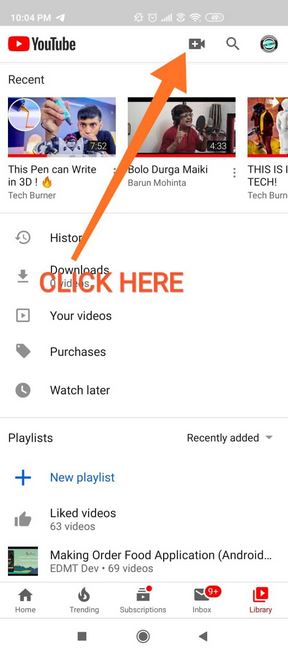This screenshot illustrates the YouTube mobile app interface on a smartphone. 

In the upper left-hand corner, the recognizable YouTube logo is prominently displayed, depicted as a red box with a white play button in the center. On the upper right-hand corner, three icons are visible: a camera, a magnifying glass (search icon), and a user profile icon represented by a circle with a green center. The camera icon is highlighted with a large orange arrow pointing towards it, accompanied by bold capital letters in orange urging users to "CLICK HERE."

Beneath the header, under the "Recent" section, three video thumbnails are partially visible. The first video thumbnail features a man holding an object, with the title "This Pen Can Write" by TechBurner. The second video thumbnail shows a man gesturing with his hands raised, titled "Bolo Durga Maiki Barun Mohinda." The third video’s thumbnail is cut off, but the title begins with "This is Tech."

Further down, a menu showcasing different features of the app is present, followed by a list of playlists. Two playlists are immediately visible: "Liked Videos" and "Making Order Food Application Android."